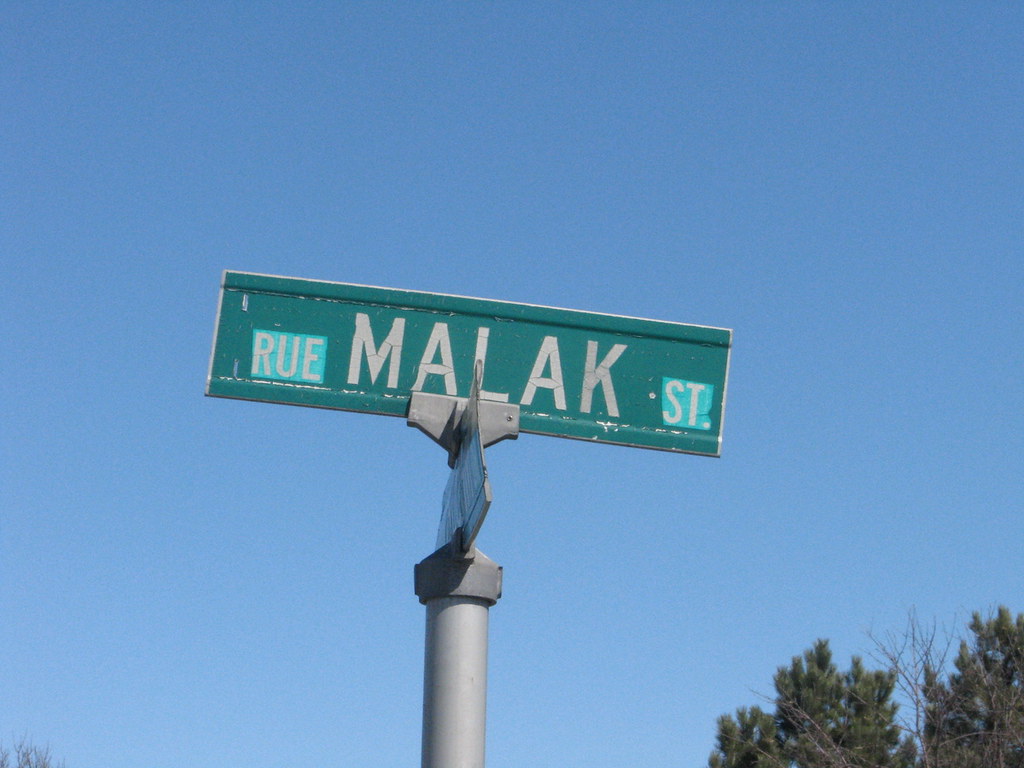This photograph captures a close-up of a slightly weathered green street sign that reads "Malak Street" in bold white text. The sign, mounted on a silver pole, shows signs of age with white markings and wear. The background features a clear, deep blue midday sky without clouds. To the bottom right of the frame, the tops of green trees are visible, along with a leafless tree's distinctive bare branches adding contrast to the greenery. The combination of the clear sky and the surrounding natural elements highlights the street sign as the central point of focus.